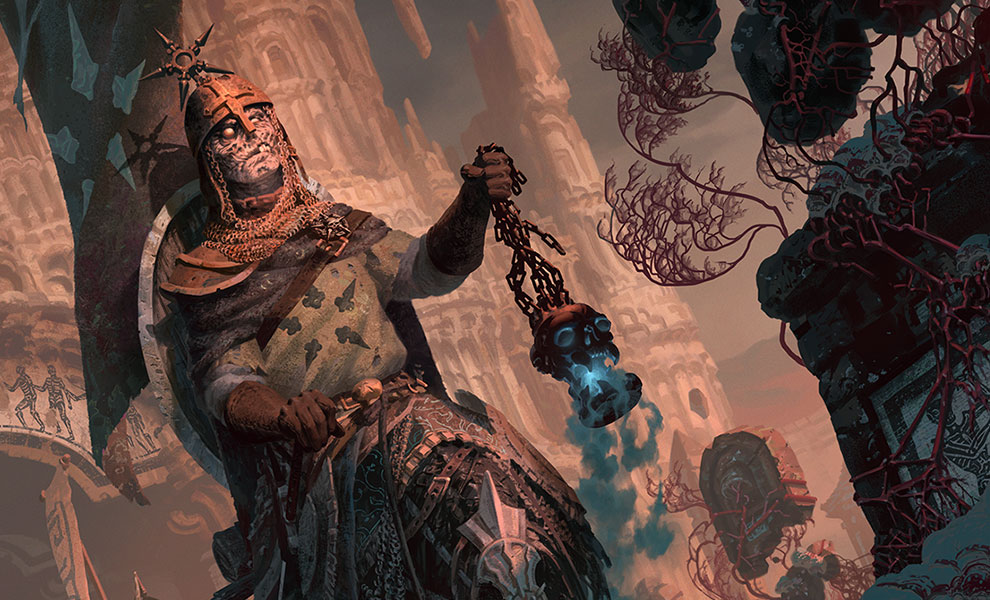The image is a cartoon-style computer-generated painting set outdoors, with the sky visible in the background. The central figure appears to be a monstrous, zombie-like soldier reminiscent of a knight from the Crusades. His face is severely distorted and deteriorating, highlighted by missing teeth and mismatched eyes, with the left eye being larger than the right. He wears a metal helmet adorned with a star on top and has a distinctive bar covering his nose. 

His attire includes dark brown gloves and a leather belt strapped across his shoulders. Around his neck is a chain, and in his left hand, he holds a gruesome lantern shaped like a skull, which emits an eerie blue light and has chains flowing from it, resembling Medusa's hair. In his right hand, he grasps what appears to be a sword handle. The background features a large, beige castle with skeletal designs faintly visible on its mid-left side, adding to the overall eerie and medieval ambiance of the scene.